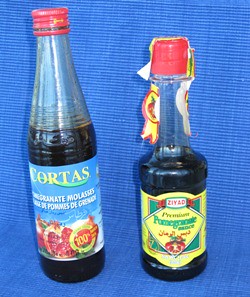This photograph captures two glass bottles filled with a dark, opaque liquid resembling soy sauce. Due to the image's blurriness and small size, the text on the labels is unreadable. The bottle on the left stands taller, adorned with a blue label featuring white lettering and an image that seems to depict a round fruit. It is topped with a red cap. The bottle on the right is shorter and rounder in shape, with a red cap that has a yellow safety sticker, which appears to be broken. Its label is predominantly yellow with green corners and accents of red. Both bottles are positioned against a blue background.